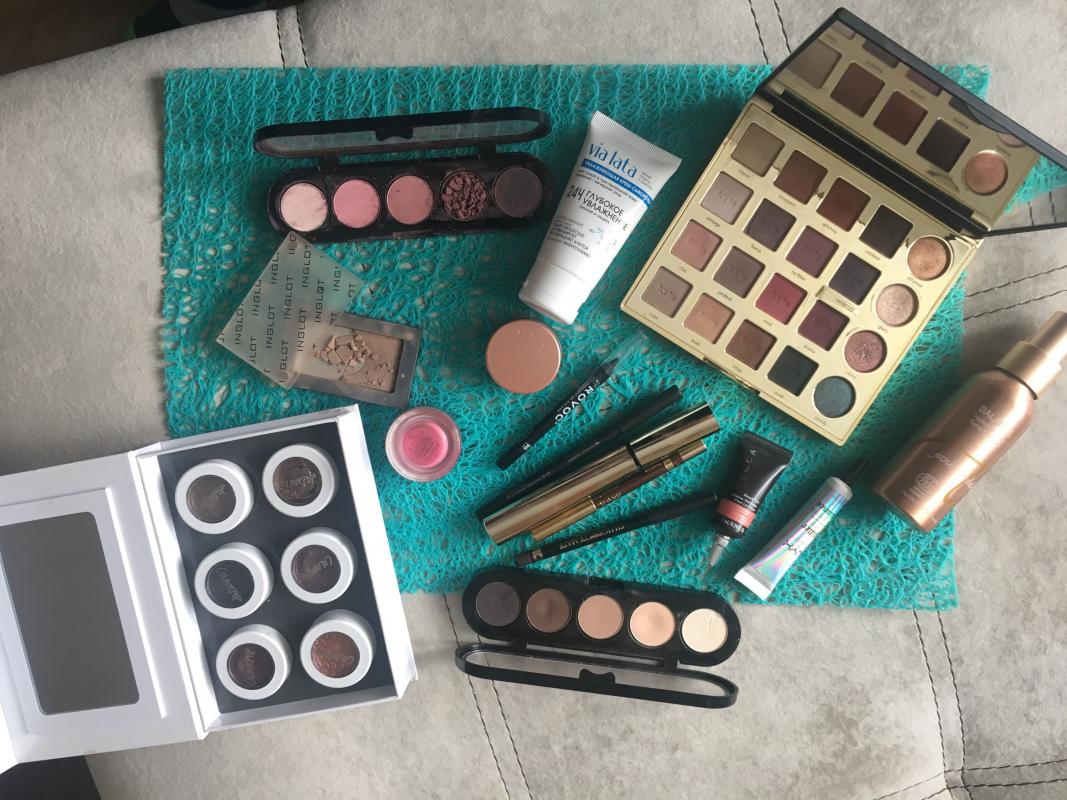This overhead photograph captures an array of makeup items meticulously organized on a vibrant turquoise, lacy doily, laid atop a light gray fabric surface, likely an ottoman or couch cushion. The doily's intricate, translucent texture contrasts with the cushion's visible stitching and pulled-in fabric details, creating a visually rich background. 

In the bottom left, a white makeup palette with an open lid reveals a rectangular mirror and six small jars containing various dark eyeshadow shades. Above it, a petite black-bordered blush case is open, showcasing brown blush dust hinting at frequent use. A white lid partially overlaps this section.

Towards the top left, a large oval palette with five colors sits open within its black case. A small white squeeze tube labeled "Violetta" in blue text lies angled to the right in the top right corner of the image.

Dominating the top right, a sizable makeup palette features five rows of four different colors, complemented by four round pots of color along its gold-backgrounded right side, encased in black. Below this, an assortment of mascaras, eyeliners, and lip liners are neatly arranged towards the center-bottom of the image.

This detailed arrangement of makeup items against contrasting textures and colors creates an inviting, well-composed visual narrative.